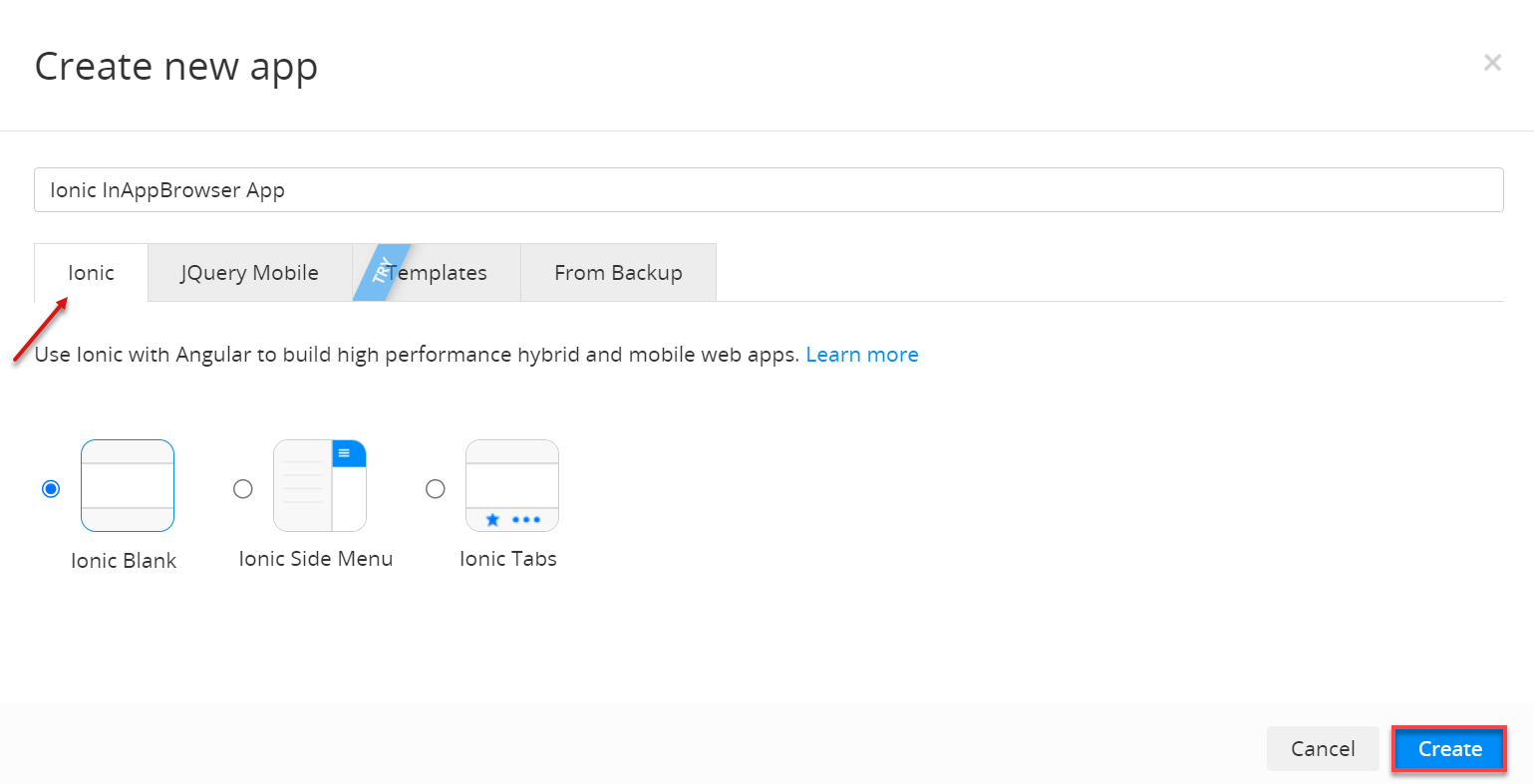The image captures a computer screen displaying the "Create New App" interface of a development platform. Centrally positioned is a faint gray line followed by a long, skinny text field where "Ionic in-app browser APP" is typed. Below this text field, the word "Ionic" is prominently displayed in two places: once alone in capital letters (I-O-N-I-C) and once with a small, skinny arrow pointing to it from the left and angled slightly upwards. Beside "Ionic," the term "jQuery Mobile" is visible under the section labeled "Templates," which also includes an option titled "From Backup."

Scrolling further down, there's a brief informative sentence stating, "Use Ionic with Angular to build high-performance hybrid and mobile web apps." This sentence is followed by a "Learn More" link, highlighted in blue. Below that, there are template options listed as "Ionic Blank," "Ionic Side Menu," and "Ionic Tabs." The "Ionic Blank" option is selected, indicated by a blue dot next to it.

At the bottom of the screen is a red rectangle enclosing the word "Create," with the button itself being a blue box.